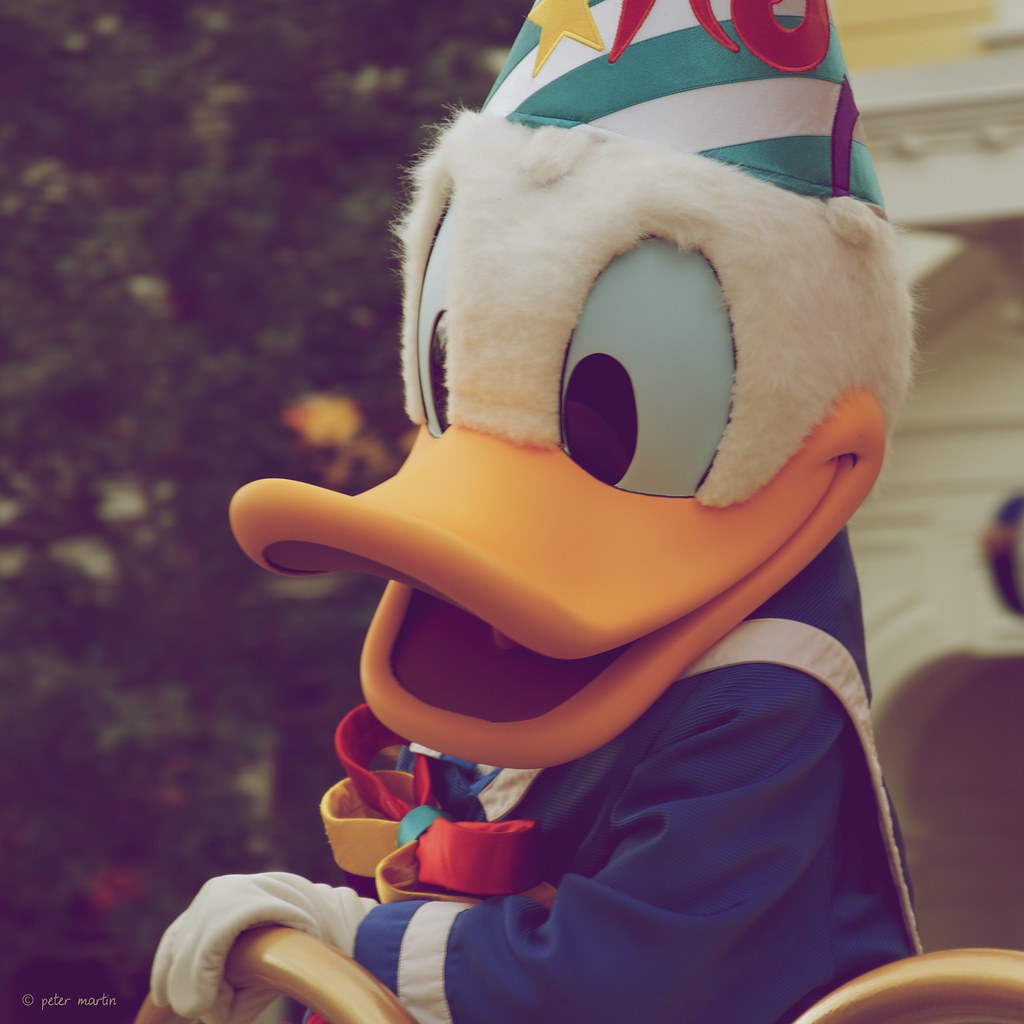This photograph depicts a close-up shot of a Donald Duck mascot, likely taken at a Disneyland or Disney World event. The mascot is dressed in a classic blue sailor outfit with white gloves, which is consistent with the character's traditional attire. Donald Duck's head is covered with a fluffy white fur, and he has a large yellow beak that appears to be smiling. The eyes are big and colored with an eggshell blue hue.

Donald Duck is also wearing a distinctive hat, which resembles a teal blue and white-striped party hat with red and purple accents and a star. At the neck, he sports a decorative bow tie or ribbon, which is made out of fabric and features gold and red ribbons with a light blue center. He has one hand resting on a gold railing, suggesting he is part of a Disneyland parade or event. 

The background of the image is blurred, showing trees on the left and what appears to be a castle structure on the right. In the lower left corner of the image, there is a "© Peter Martin" watermark.